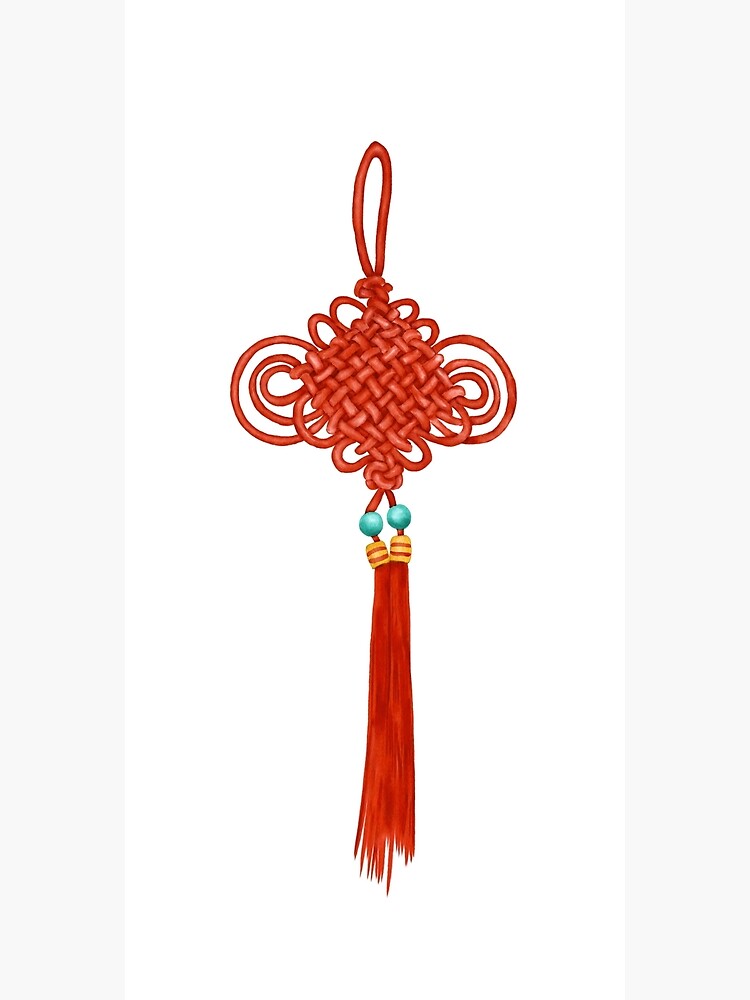This image depicts a detailed watercolor painting of a traditional Chinese Knot, set against a plain white background. The knot is predominantly red, featuring an intricately braided design at the top, with ornate loops adding to its decorative allure. A prominent hanging loop crowns the knot, designed for display purposes. Below the knot, two distinct blue beads, described as turquoise-like or jade-colored, introduce a vibrant contrast. These beads are followed by smaller red and yellow beads, enhancing the overall intricate design. Extending from these beads are two long red tassels, completing the knot's traditional aesthetic. The artwork, which captures this emblematic Asian cultural artifact believed to bring good luck, showcases the use of delicate watercolor techniques, making the colors and details stand out vividly against the white backdrop.